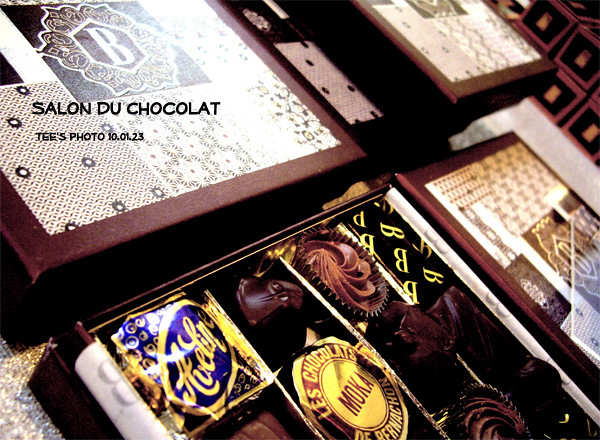The photo captures an elegantly arranged collection of chocolate boxes, each exuding a sense of luxury and sophistication. At the forefront, one box stands out with its lid removed, displaying an assortment of exquisite chocolates and candies nestled in their respective slots. These treats vary in appearance: some are wrapped in shimmering gold or purple foil, while others sit in crinkly brown paper cups, showcasing intricate designs such as swirls, fudge, or chocolate-covered nuggets. Notably, several of the candies are adorned with fancy labels, including "Mocha" and a prominent letter "B," suggesting the branding of the chocolatier. Surrounding this open box are three more unopened, elaborately decorated boxes, featuring delicate embroidered patterns. The entire scene is artistically angled, with a visible watermark on the left side that reads "Salon du Chocolat, T's Photo, 10.01.23," indicating the source and date of the image.